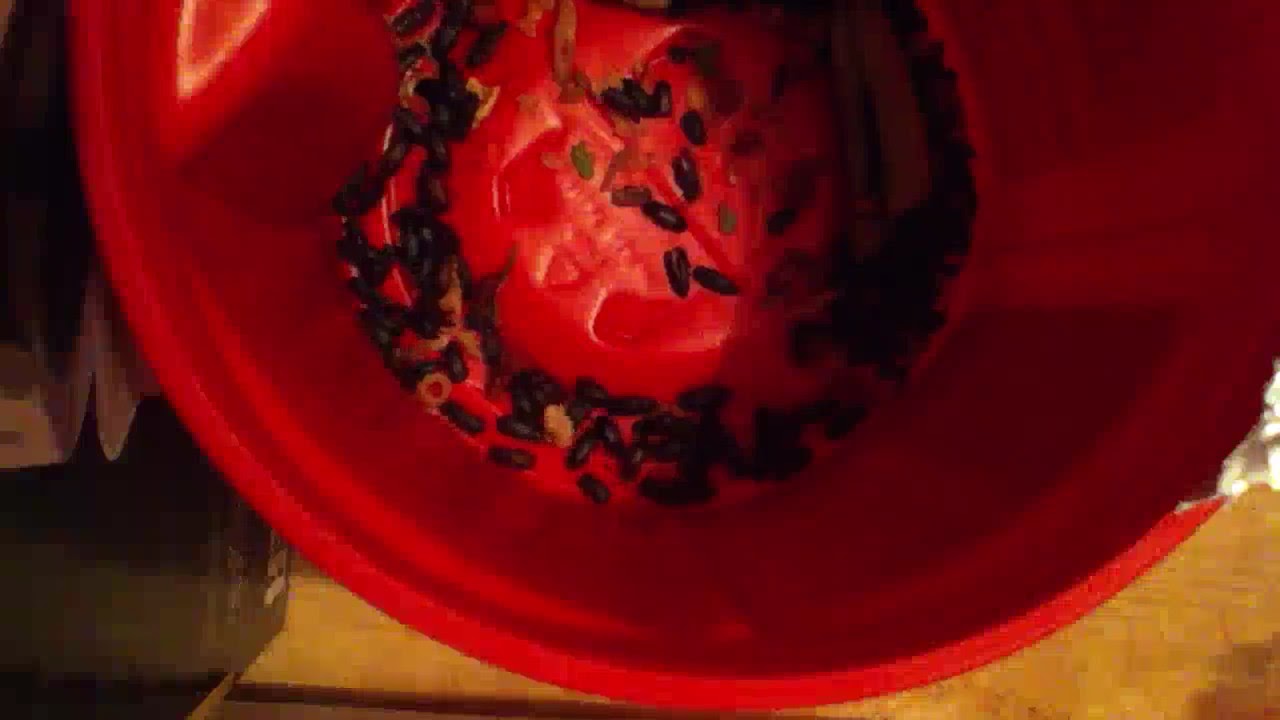This photo captures a top-down view of a red bucket, revealing about half of its interior. The bucket contains dozens of oval-shaped objects, mostly dark black, which could be seeds or insects. Some light brown, smaller oval shapes are also scattered among them. Most of these objects are clustered around the edges, forming a circle, with a few dispersed in the center, exposing the bottom of the bucket. The bucket, possibly made of styrofoam, features a significant indent or tear on the top left, exposing a powdery material underneath. The right side of the bucket appears to have some string or labels attached. The bucket is placed on a wooden surface, and in the bottom left corner of the photo, there is an indistinct dark, square-shaped object.